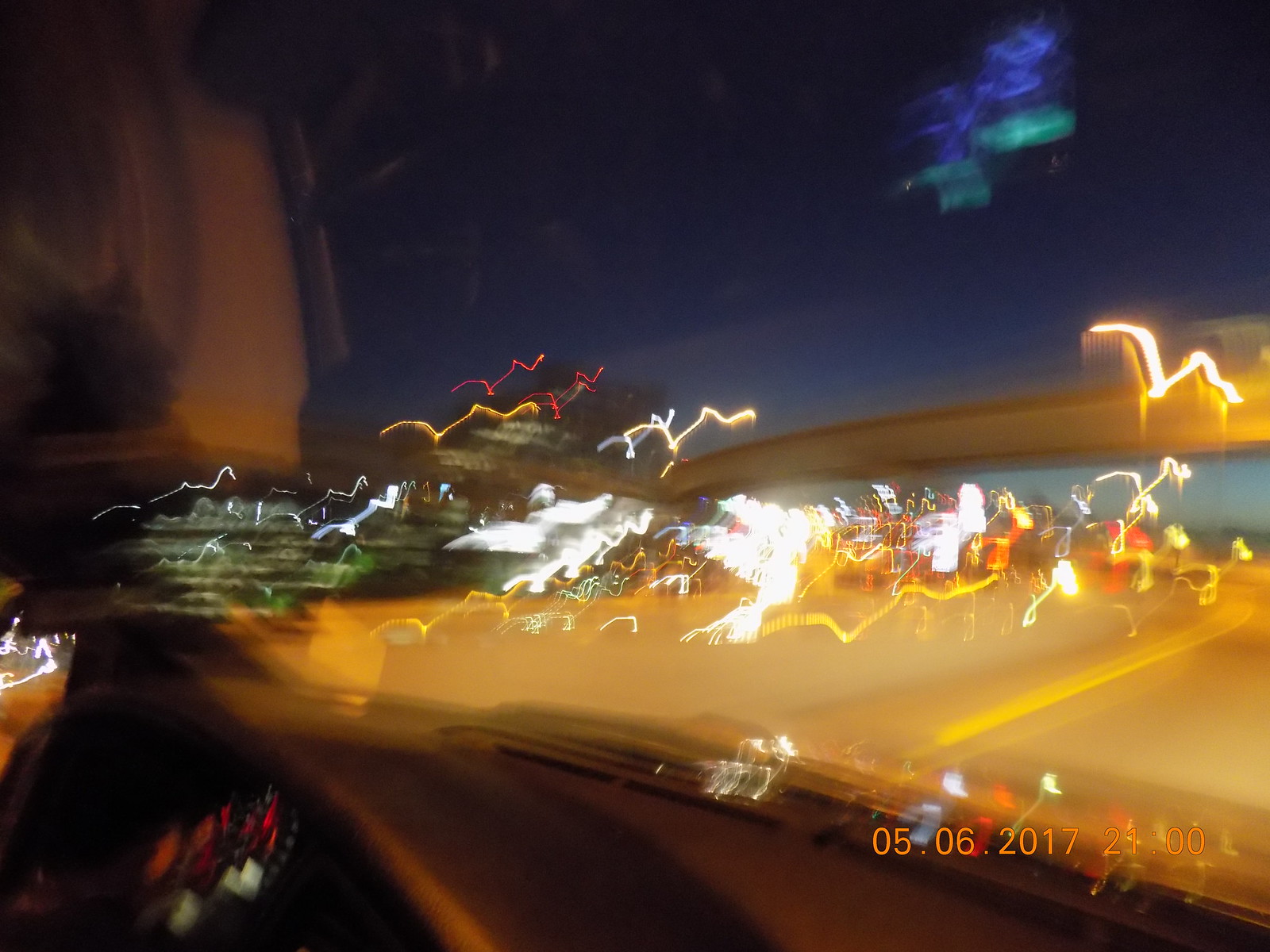In this rectangular photograph, we observe a slightly blurry image with visible editing effects overlaid. The vantage point is from within a vehicle, peering out through the windshield. The scene beyond the windshield depicts a distant cityscape on the left horizon, suggesting a mix of urban structures visible in the far distance. The foreground displays a road, marked by a yellow dividing line down the center, while a gray divider wall is present on the left side of the roadway.

In the lower right corner of the image, an orange text indicates the date "5-6-2017" and the time "2100". The windshield catches light, creating prism-like glints that refract into squiggly lines of red, yellow, and white streaks across the image, adding a surreal touch to the composition.